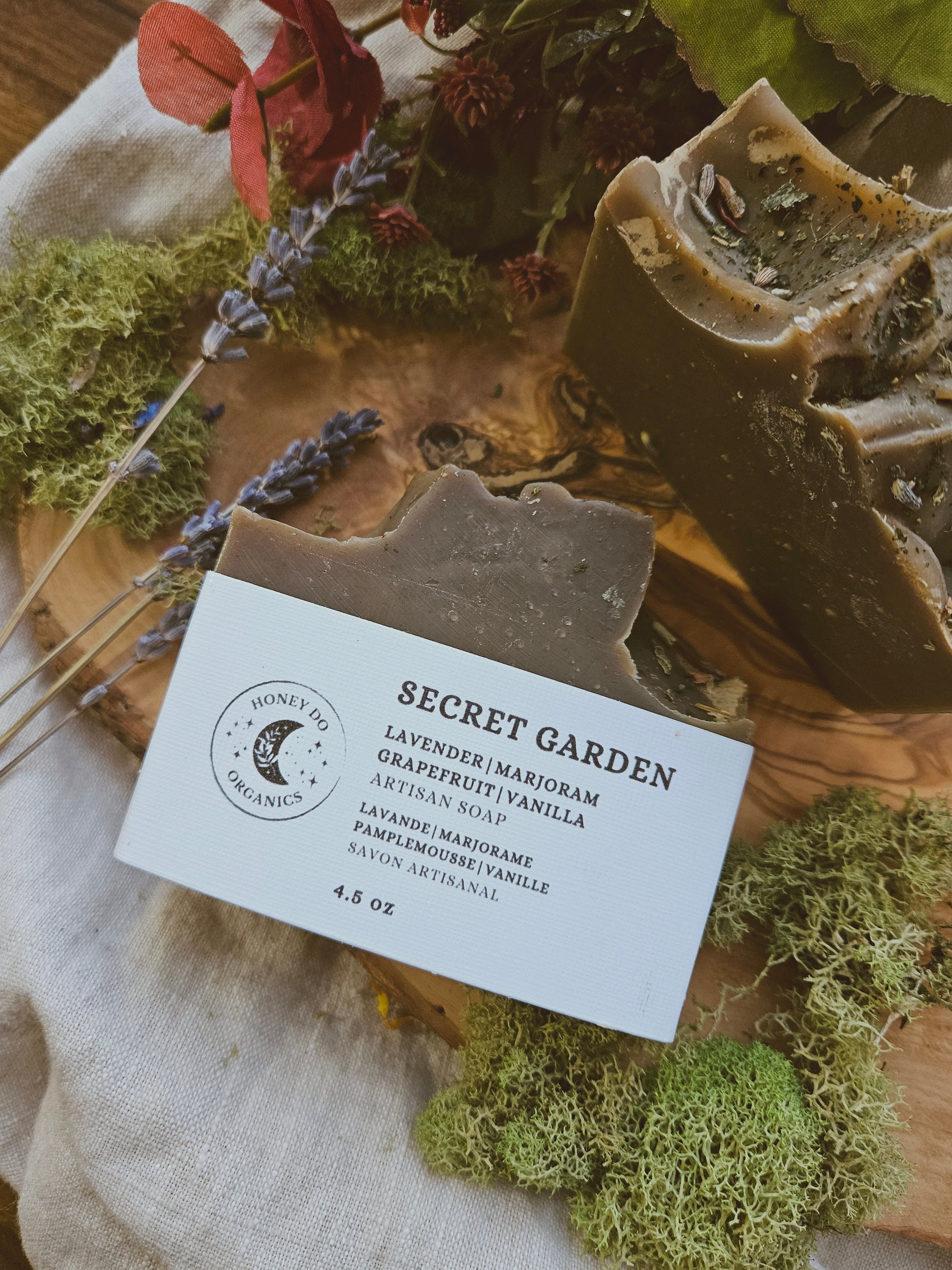The image is an advertisement for an artisanal soap branded by Secret Garden, produced by Honeydew Organics. The soap, which weighs 4.5 ounces, features an intriguing blend of lavender, grapefruit, vanilla, and marjoram. This organic soap is depicted as a brown, jagged bar dusted with various spices, and positioned beneath a white business card also displaying a French translation. The card, featuring dark gray text, has the Secret Garden logo alongside a circular Honeydew Organics logo with a moon in the center. The presentation is set against a rustic backdrop: the soap rests on a walnut cross-section of a stump, adorned with green moss, red and green leaves, and purple flowers. This natural display sits atop a white, slightly yellowish linen tablecloth.